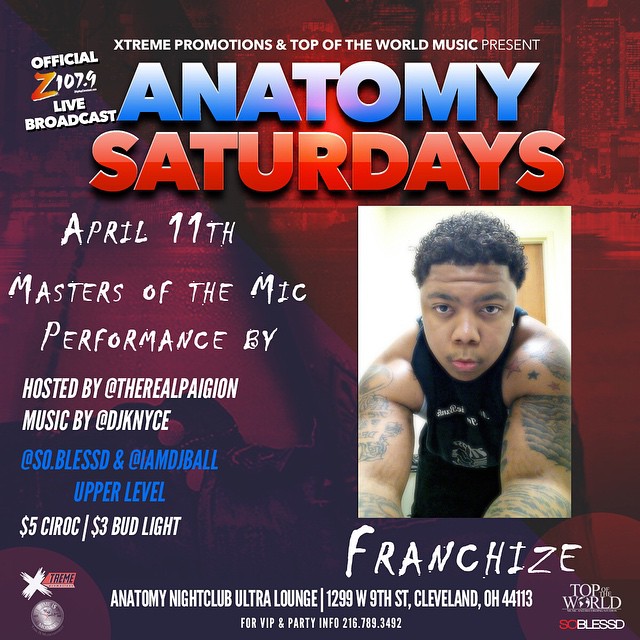The poster promotes “Anatomy Saturdays” at Anatomy Nightclub Ultra Lounge, located at 1299 West 9th Street, Cleveland, Ohio 44113. At the very top in white letters, it announces "Extreme Promotions and Top of the World Music Present Anatomy Saturdays." The word "Anatomy" is prominently displayed in blue, and "Saturdays" in red. On the left side, it features "Official Z107.9 Live Broadcast," with the Z's highlighted in orange and yellow. Below this, in white, it states "April 11th, Masters of the Mic Performance by Franchise," accompanied by a picture of the performer Franchise, who is Afro-American, looking into the camera, wearing a black tank top with white writing. His name, "Franchise," is spelled out beneath the image in white. The event is hosted by @TheRealPaigion and music is provided by DJ KNYCE, with additional mentions of DJs like @SoBlessed and @IAmDJBall. It also highlights the drink specials: $5 Ciroc and $3 Bud Light. The bottom of the poster provides contact information for VIP and party details: 216-789-3492. Logos for “Top of the World” and “So Blessed” are present in the corners.